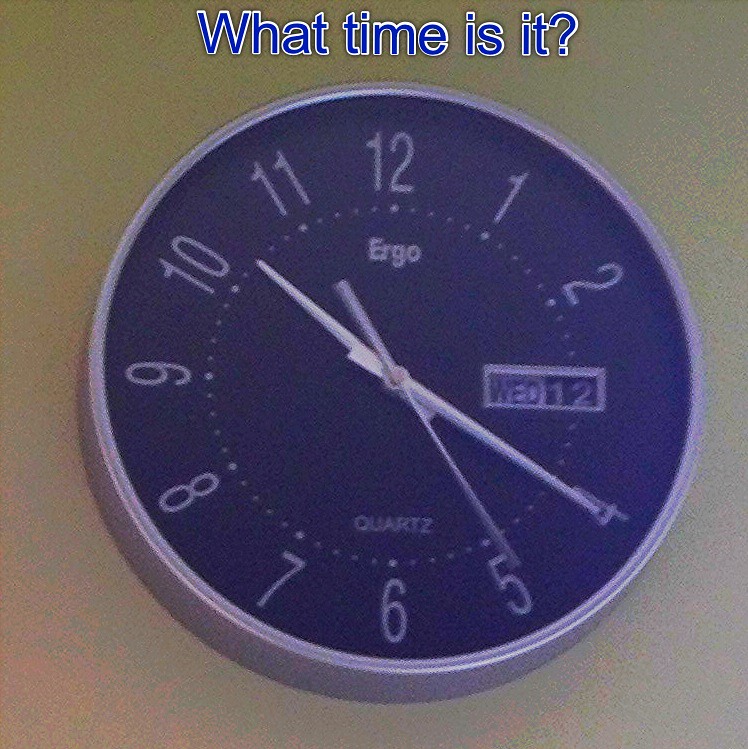The image displays a grainy, out-of-focus, brown background with a clock prominently featured in the center. The clock face, which is primarily black, shows blue text at the top reading "What time is it?" The numerical markers around the clock display the hours in an unconventional format: the numbers "2" and "3" are missing, but the rest of the numbers from "1" to "12" are present. Surrounding the center of the clock are small dots positioned where the numerical markers usually are.

At the top of the clock face is the word "Ergo" in white text, while the bottom reads "Quartz" in similar lettering. The hour hand points between the numbers 10 and 11, the minute hand is at the 4, and the second hand is at the 5. There is also a small window on the right side of the clock's face that displays the day and date: "Wednesday" in black text on a white background, and "12" in white text on a black background.

The clock is encased in a silver frame and mounted on a wall. A shadow is cast on the wall below the clock, adding depth to the scene.